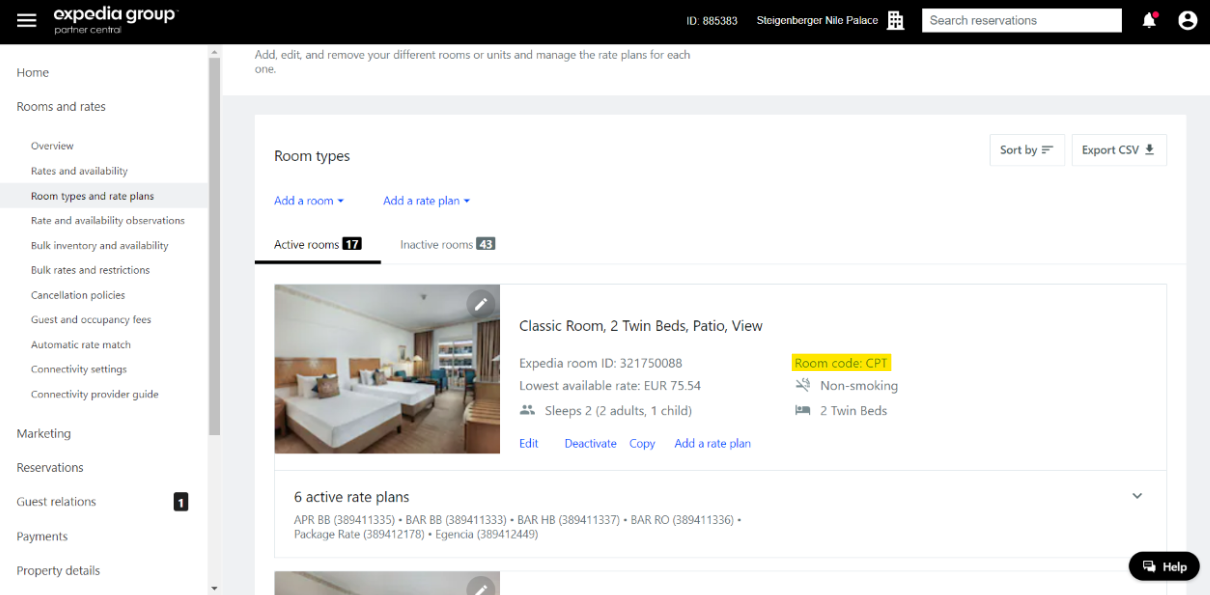The image depicts a user interface from Expedia Group's hotel booking management system. At the top, the page prominently displays the "Expedia Group" logo, indicating that this is part of the Expedia travel website. On the left-hand side, a comprehensive menu lists various options for managing hotel bookings, including "Rooms and Rates," "Overview," "Rates and Availability," "Room Types and Rate Plans," "Rate and Availability Observations," "Bulk Inventory and Availability," "Bulk Rates and Restrictions," "Cancellation Policies," "Guest and Occupancy Fees," "Automatic Rate Match," "Connectivity Settings," "Connectivity Provider Guide," "Marketing," "Reservations," "Guest Relations," "Payments," and "Property Details."

On the right side of the interface, there is a section labeled "Room Types," specifically focusing on "Active Rooms." Here, the viewer sees an example of a room available for booking, described as a "Classic Room" featuring "Two Twin Beds" with a "Patio View." The visual representation of the room shows two neatly made beds, a desk, and a table, providing potential guests with a clear idea of the accommodations offered. This setup appears to be a detailed administrative tool for property managers to oversee and adjust their listings on Expedia.